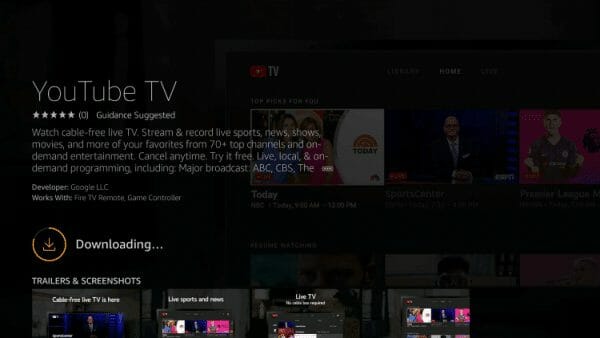A screenshot taken from a computer displays a YouTube TV webpage, predominantly dark with a black background. The user seems to be in the process of downloading YouTube TV, as an icon indicates the download is approximately 25% complete. At the top of the page, the header reads "YouTube TV," accompanied by a rating system showing five fully-filled stars and the note "Guidance Suggested." 

The main text promotes the service with the message: "Watch cable-free live TV, stream and record live sports, news, shows, movies, and more of your favorites from 70+ top channels and on-demand entertainment. Cancel anytime. Try it free." 

Additional information at the bottom highlights features like "Live local and on-demand programming including major broadcast ABC, CBS, Th..." though the text appears cut off. Below this, there are clickable boxes labeled "Trailers" and "Screenshots," with one clearly marked "Live TV." The rest of the webpage remains dark.